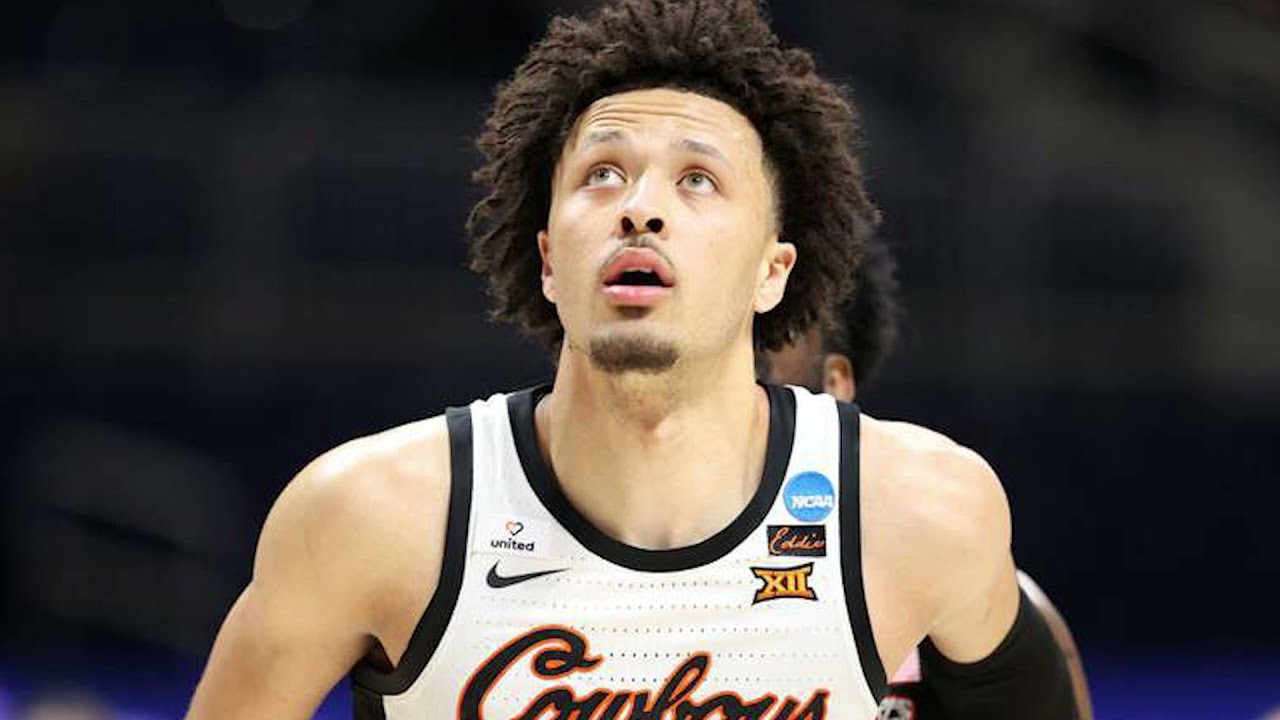This detailed close-up image captures a Cleveland Cavaliers basketball player during an intense moment of a game. The player is wearing a white jersey adorned with orange, black, blue, and yellow text and logos, including the NCAA logo on the top right and a gold "XII" lower down. The Nike checkmark is visible on the left side, along with a multicolored heart above the word "UNITED" in black font. With bushy black hair, a slight beard, and mustache, the player looks upwards, possibly at the scoreboard or a replay. His mouth is open, reflecting his focus and intensity. The background is heavily blurred, obscuring the details and only showing part of another person’s left ear and hair. There's also a blue board visible along the lower horizontal axis of the photo. The player's upward gaze suggests he might be tracking the ball or observing a play unfold.